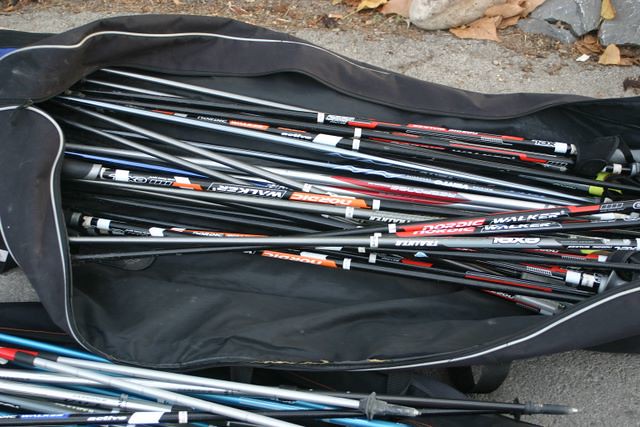The image captures an outdoor scene with a black nylon duffel bag prominently placed on an asphalt surface. The bag, which bears the brand name "Walker," features white trim and is open, revealing its contents. Inside the bag are numerous poles that have been disassembled. These poles, which exhibit a variety of colors including black, gray, white, blue, orange, red, and yellow, could be interpreted as fishing poles, walking poles, or even skiing poles, though the exact type is unclear due to the lack of visible tips or ends. Scattered on the ground beside the bag are additional pole pieces, creating a sense of disarray. At the top of the photo, an area of dirt with dry grass, brown leaves, and rocks adds to the rustic, outdoor ambiance.